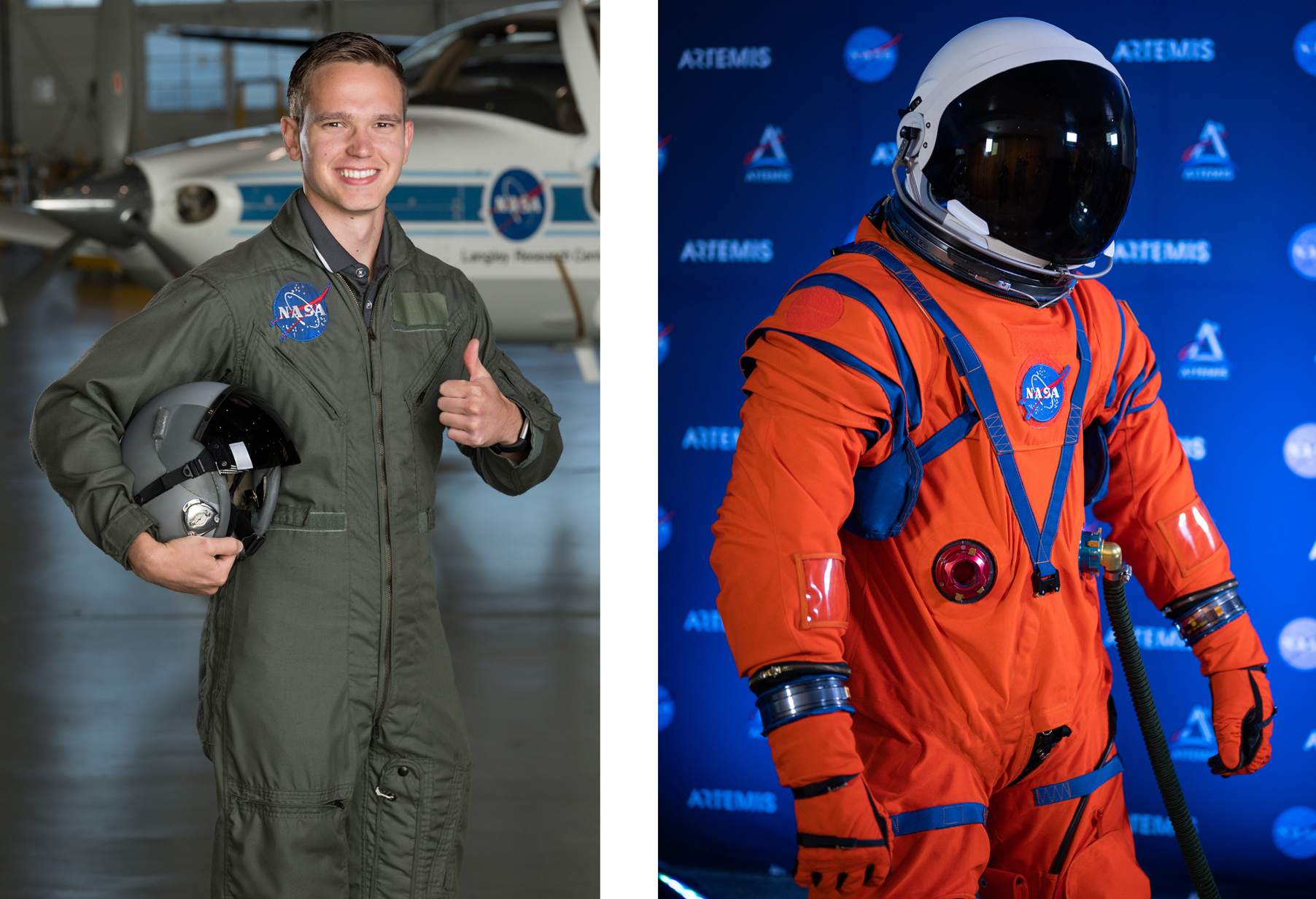The image consists of two side-by-side photos of astronauts. On the left, an astronaut, a white man, is seen wearing an olive green jumpsuit with a NASA logo. He is holding a helmet under his left arm and giving a thumbs-up with his right hand while looking directly at the camera. A NASA plane is visible in the background behind him. On the right, another image shows an astronaut in a bright orange spacesuit with blue Velcro straps and a NASA logo. This astronaut is wearing a full space helmet with a white back and dark front, standing against a blue step-and-repeat backdrop featuring the Artemis mission logo and the NASA logo. Although the helmet obscures the face, there is an implication that these two images might depict the same astronaut in different gear.